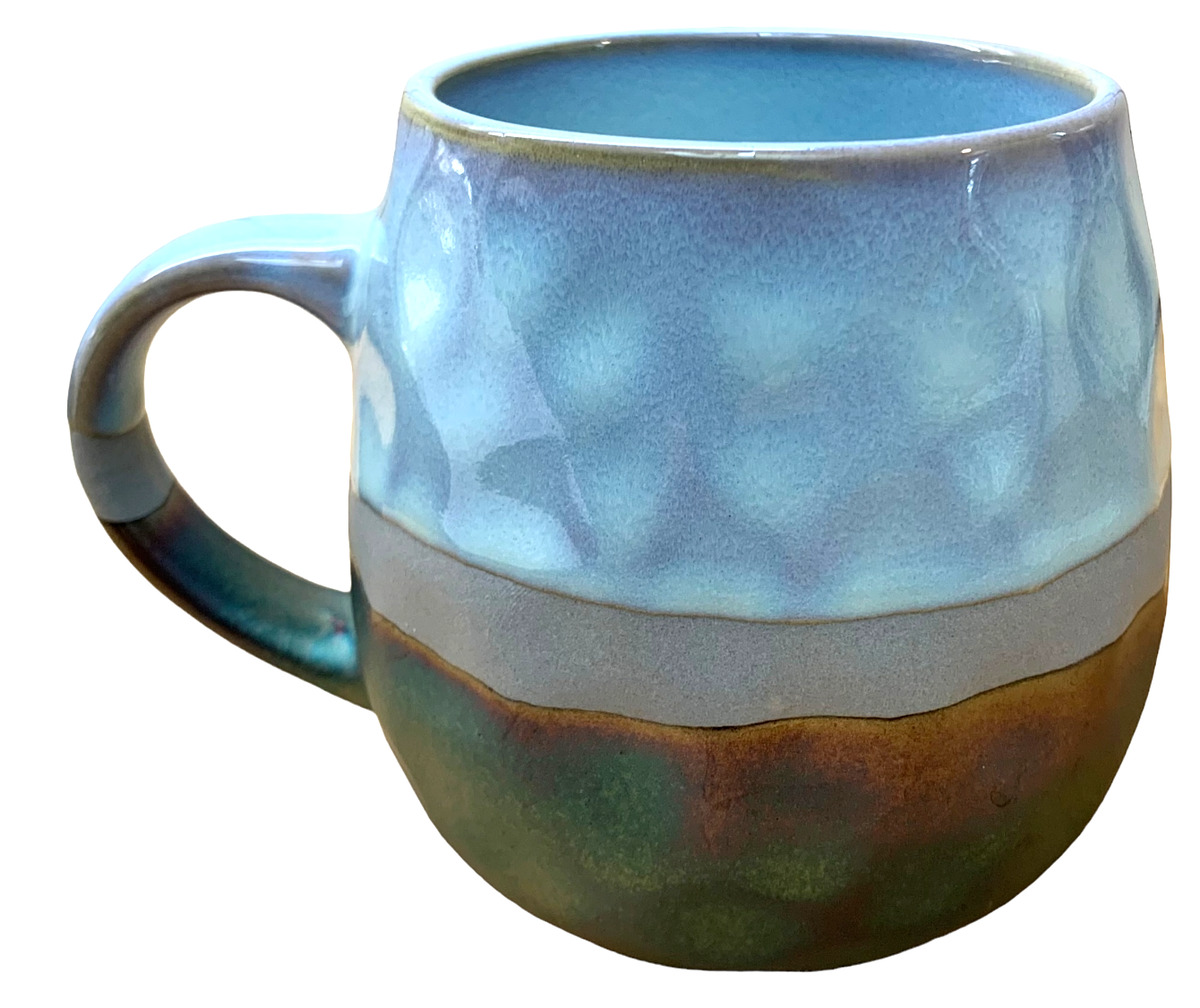This close-up, detailed photograph showcases a large, glossy ceramic coffee mug with a bulbous, hand-crafted appearance. The image, set against a solid white background, emphasizes the mug's rich, multi-colored design. Starting from the bottom, the mug features a blend of dark green and earthy brown colors, which rise to meet a gray stripe encircling the middle. The upper half of the mug transitions into a gradient of blues—beginning with a darker blue at the top and fading into lighter blue hues. The mug's rim also exhibits a grayish tone. The texture of the mug is gently dimpled, enhancing its handmade charm. The handle, situated on the left side, mirrors the mug's color scheme: light blue at the top, gray in the middle, and blending into dark green and brown at the bottom. The interior of the top part of the mug is also light blue, maintaining harmony with its vivid exterior.